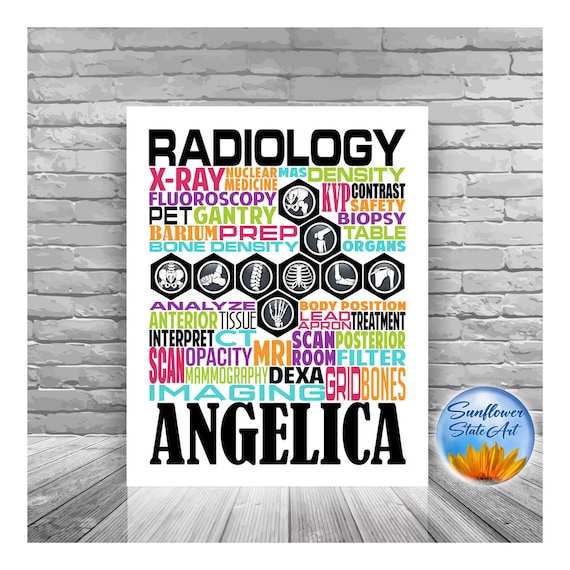The image showcases a visually striking poster, possibly computer-generated, set against a gray painted brick wall and a matching gray wood-textured floor, creating a monochrome ambiance. The poster itself rests upon the floor and features a diverse array of radiology-related terms in various vibrant colors including shades of pink, blue, green, purple, black, gold, orange, and burgundy. Key terms prominently displayed include "Radiology" at the top and "Angelica" at the bottom, both in bold black font but in distinct styles. Numerous medical terms like "x-ray," "nuclear medicine," "mass density," "fluoroscopy," "KVP," "contrast safety," "biopsy," "table," "organs," "barium prep," "bone density," "scan," "MRI," and "mammography" are scattered across the poster in a variety of sizes and orientations, creating a word art effect. Additionally, the poster features black hexagons, each containing a white outlined circle with bone structure illustrations inside. In the bottom right corner of the image is the logo for Sunflower State Art: a blue circle with sunflower petals at the bottom and the text "Sunflower State Art" in a darker blue hue.